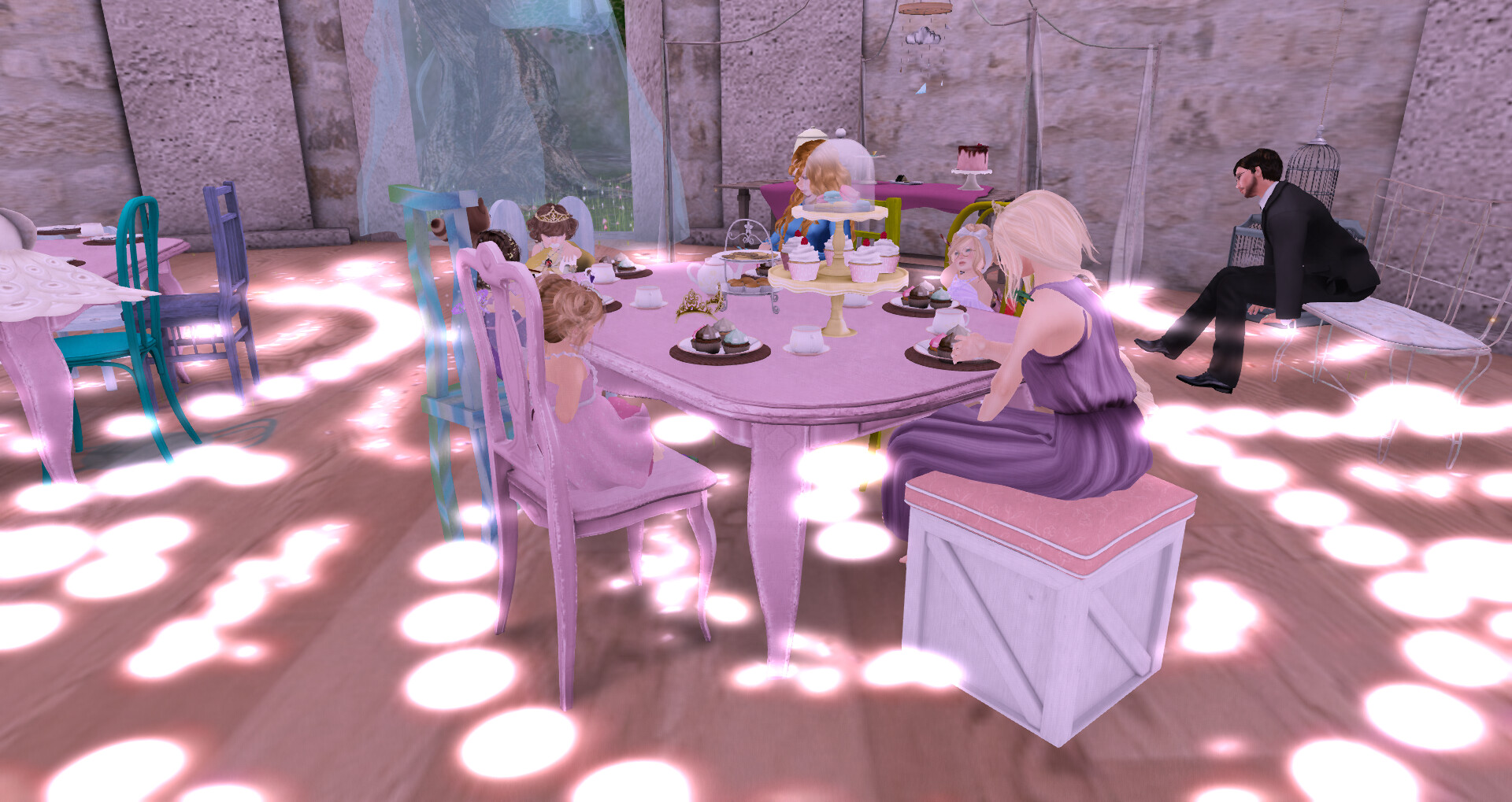The scene is a digitally rendered image resembling a setting from a game like The Sims, featuring an elegant tea party in a whimsical, dollhouse-like restaurant. The horizontal rectangular image is bathed in a pinkish-purple hue, creating a dreamy atmosphere. The background showcases a unique concrete wall with vertical rectangles that start flat on the left and curve towards the right. 

The floor is pink with white dots, and the furniture is a mix of pink, purple, and blue wood tables and chairs. At the main table, a woman and several well-dressed children, potentially three to four little girls in princess dresses (one notably wearing a gold crown), are seated. They have plates of cupcakes and a two-tiered tray of cupcakes covered with a glass dome in front of them. 

An older girl or woman in a purple dress sits on a pink-cushioned box. In the background, on the right side, a man dressed in a black suit sits on a white bench against the wall. The overall aesthetic is vibrant and playful, reminiscent of a fairytale tea time.